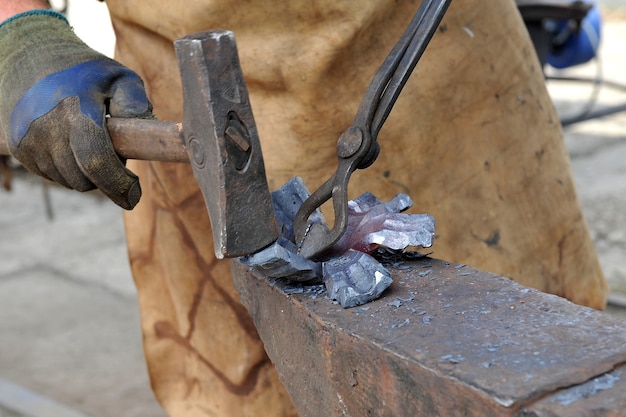The image depicts a close-up, professionally photographed scene of a blacksmith engaged in metalwork. The focus is on the blacksmith's torso and hands, which are clad in thick protective gloves—green with a blue stripe. He wears a deeply weathered brown apron with visible stains and tears, emphasizing the rugged nature of his work. The blacksmith is manipulating a piece of iron on a slim, rusting anvil, highlighted with patches of blue, possibly from oxidation or metal residues. In his right hand, he firmly grips a wooden-handled hammer, poised mid-strike. His left hand, though not fully visible, appears to wield a pair of metal tongs that securely hold the iron piece in place. The background is a neutral gray, keeping the focus squarely on the intense, tactile process of molding and shaping molten metal.